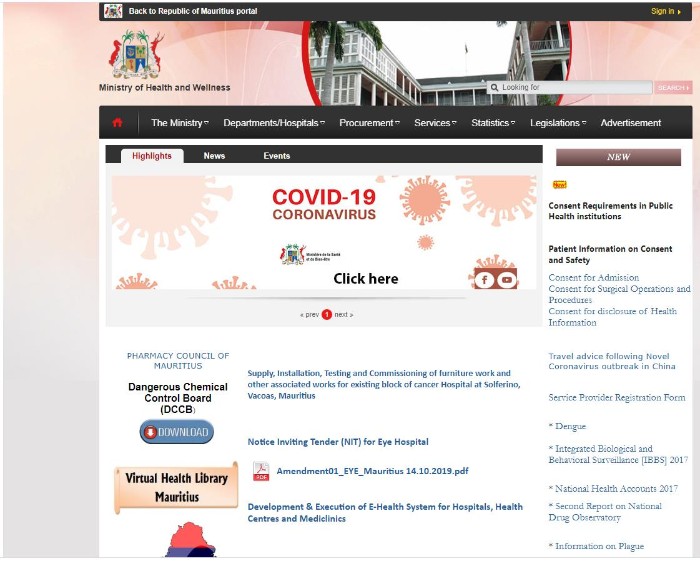This image is a detailed screenshot from a website identified as the official portal for the "Republic of Montelis." The page has a black border at the top, prominently displaying the name "Republic of Montelis." Below this, the header has a pink background and features various elements.

In the upper left-hand corner, there's an emblem that resembles a coat of arms, inscribed with "Ministry of Health and Wellness." Centrally placed within the header is an image showing just the top floor of what appears to be a large, institutional building, likely a hospital or an academic center, characterized by its gray, industrial appearance.

Directly beneath the header, a black navigational menu is organized horizontally, listing the following sections from left to right: "The Ministry," "Departments/Hospitals," "Procurement," "Services," "Statistics," "Legislation," and "Advertisement."

The main section of the webpage has a white background. Near the top and slightly to the left, there's a large graphic. The text "COVID-19" is prominently displayed in pink font, with "coronavirus" written beneath it. The rectangular graphic features schematic drawings of the coronavirus on either side, depicted like a sun with radial nodules, rendered in white.

On the right side of the page, a vertical menu is present. A brown banner at the top of this menu reads "new." The menu starts with an item titled "Consent Requirements in Public Health Institutions," followed by a detailed list of various other items.